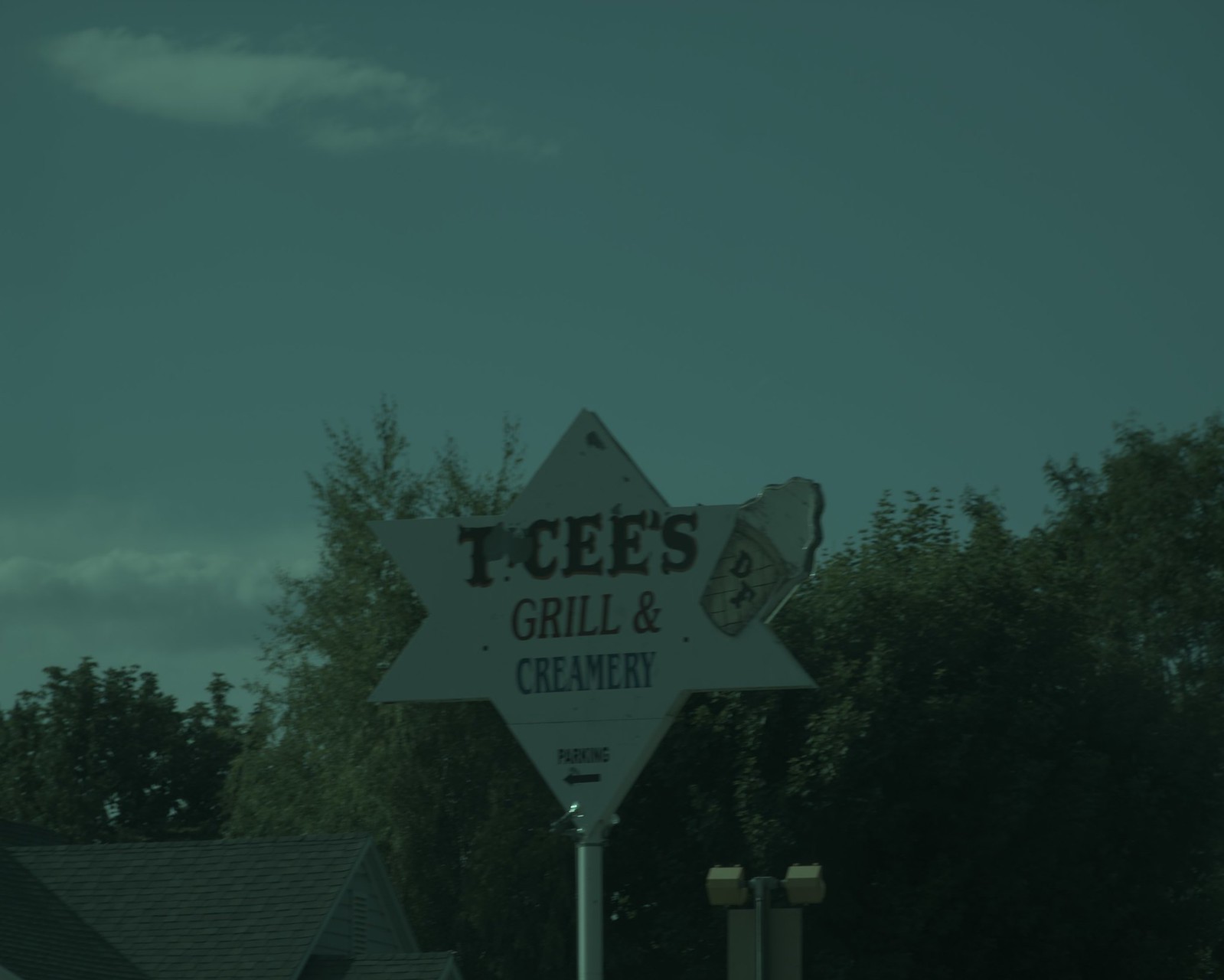The image captures an outdoor scene under a medium gray-blue sky peppered with clouds primarily at the top left and bottom left. In the mid-ground, a variety of trees fill the landscape, transitioning from shorter trees on the left to taller, lush trees of different types such as oak, pine, and evergreen as the eye moves towards the right. In the bottom left corner stands a building. The image prominently features a central pole with a star-shaped sign made of two overlapping triangles. The sign reads "Tee's Grill and Creamery" and "Parking" at the bottom, with an ice cream cone icon adorning the top.